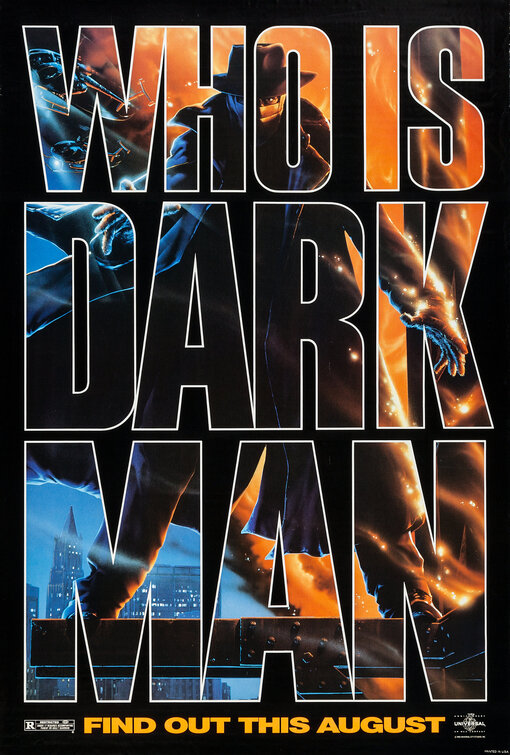In this dramatic, promotional movie poster for Sam Raimi's "Darkman," vivid elements combine to create an intense and gripping visual. The black background prominently features large, white-outlined letters making up the title "Who is Darkman." Inside these letters, you can see a striking composition: a man dressed in a black trench coat and pants, a black top hat, and a white cloth covering his face, revealing only his eyes. His dark, billowing cape and black shoes add to the enigmatic figure. Flames burst vibrantly from the right-hand side of the image, slightly burning his left arm, adding a sense of peril and action.

The man appears to be standing on the bricked frame of an unfinished building, seemingly high above a nighttime cityscape. The tops of skyscrapers with illuminated windows suggesting inhabited buildings create a dramatic backdrop. This scene, depicted in a poster that blends illustration and comic book artistry, gives the impression that Darkman is almost flying over the city.

At the bottom, promotional text in orange font reads "Find out this August," indicating the film's release date. The poster also includes essential details: a Universal Pictures logo in the bottom right corner and a "Rated R" notification in the bottom left, completing the commercial allure of this early 90s movie campaign.